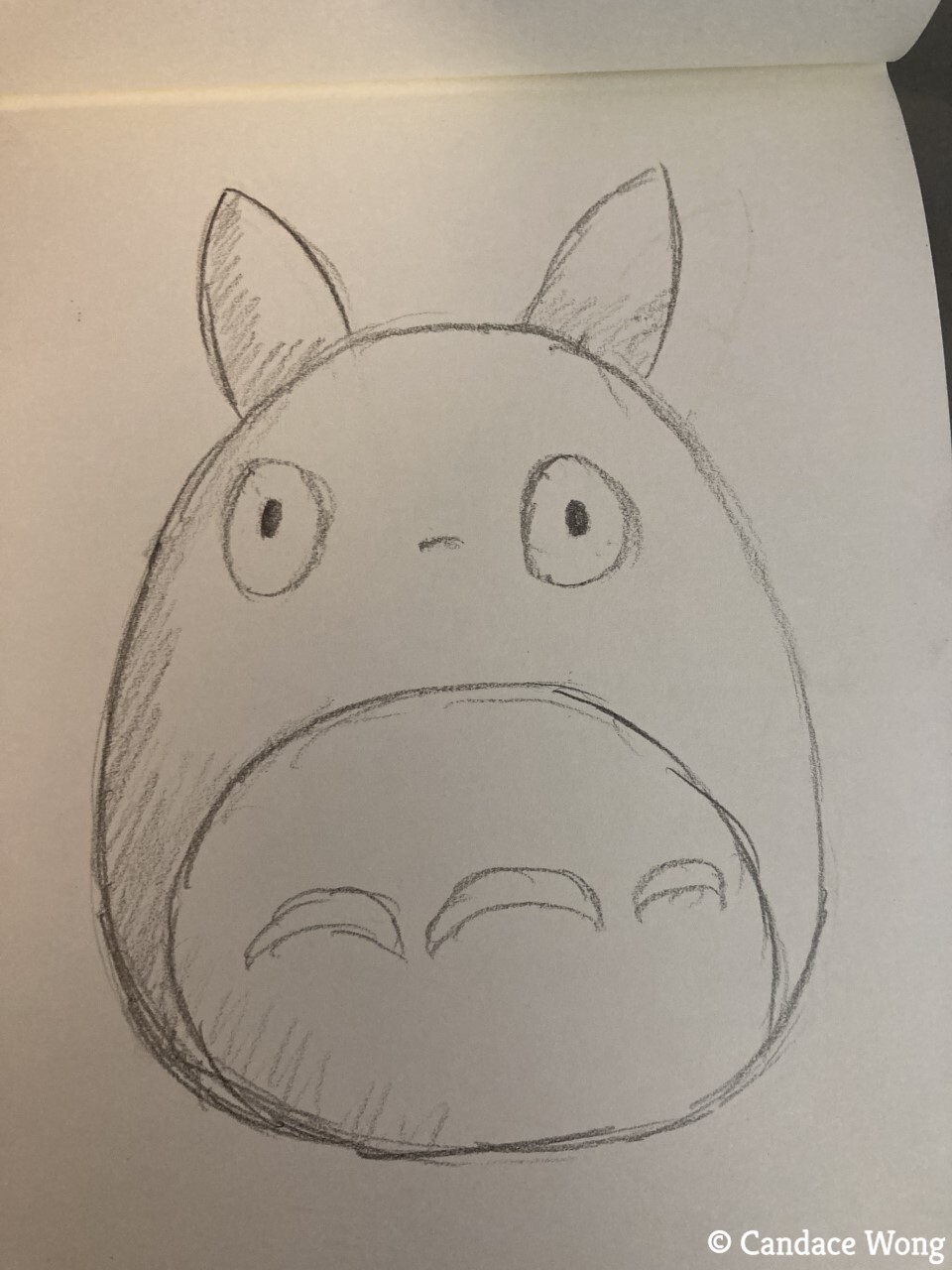This is a detailed drawing of a horse’s head on a clean white sheet of paper, captured from a frontal perspective. The horse is depicted as if it is staring directly at the viewer. The eyes are represented by two larger circles, each containing smaller, colored-in circles to suggest pupils. The horse's ears are pointed and positioned atop its head. The head itself is shaped like an elongated oval, culminating in a smaller circle at the bottom, representing the horse’s muzzle. This circle features a series of small, crescent-shaped arcs, presumably to illustrate the texture or detail of the muzzle. In the bottom right corner of the page, the artist's name, Candice Wong, is neatly inscribed in white.